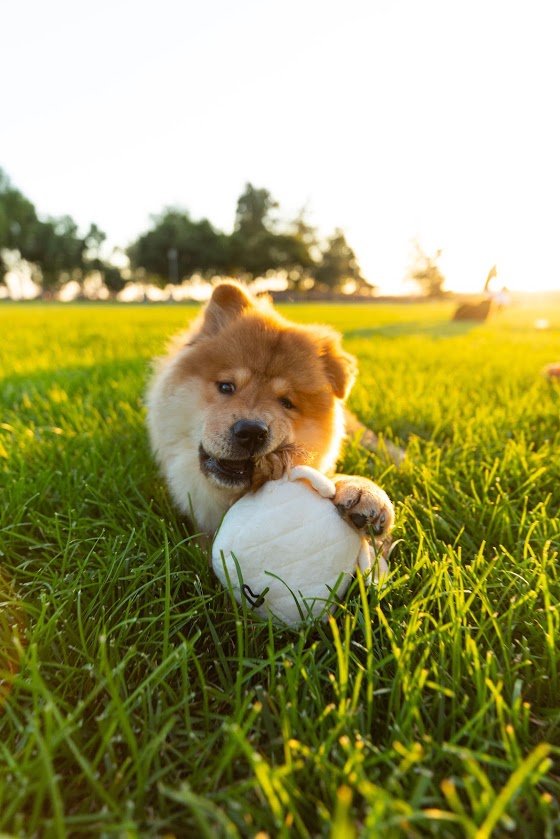The photograph captures a golden-colored, fluffy corgi lying in a lush, green field, holding a circular white stuffed animal with its left paw. The image focuses on the corgi's head, which is angled towards the camera, showing a serene and playful scene. The grassy field, likely in a park or open area, is bathed in the warm, golden light of a setting sun, casting a soft, yellowish hue over the grass, particularly on the right-hand side. In the background are blurry, vibrant green trees, and the sky above is bright white, clear, and illuminated by the sun’s rays, enhancing the tranquil atmosphere of the scene.